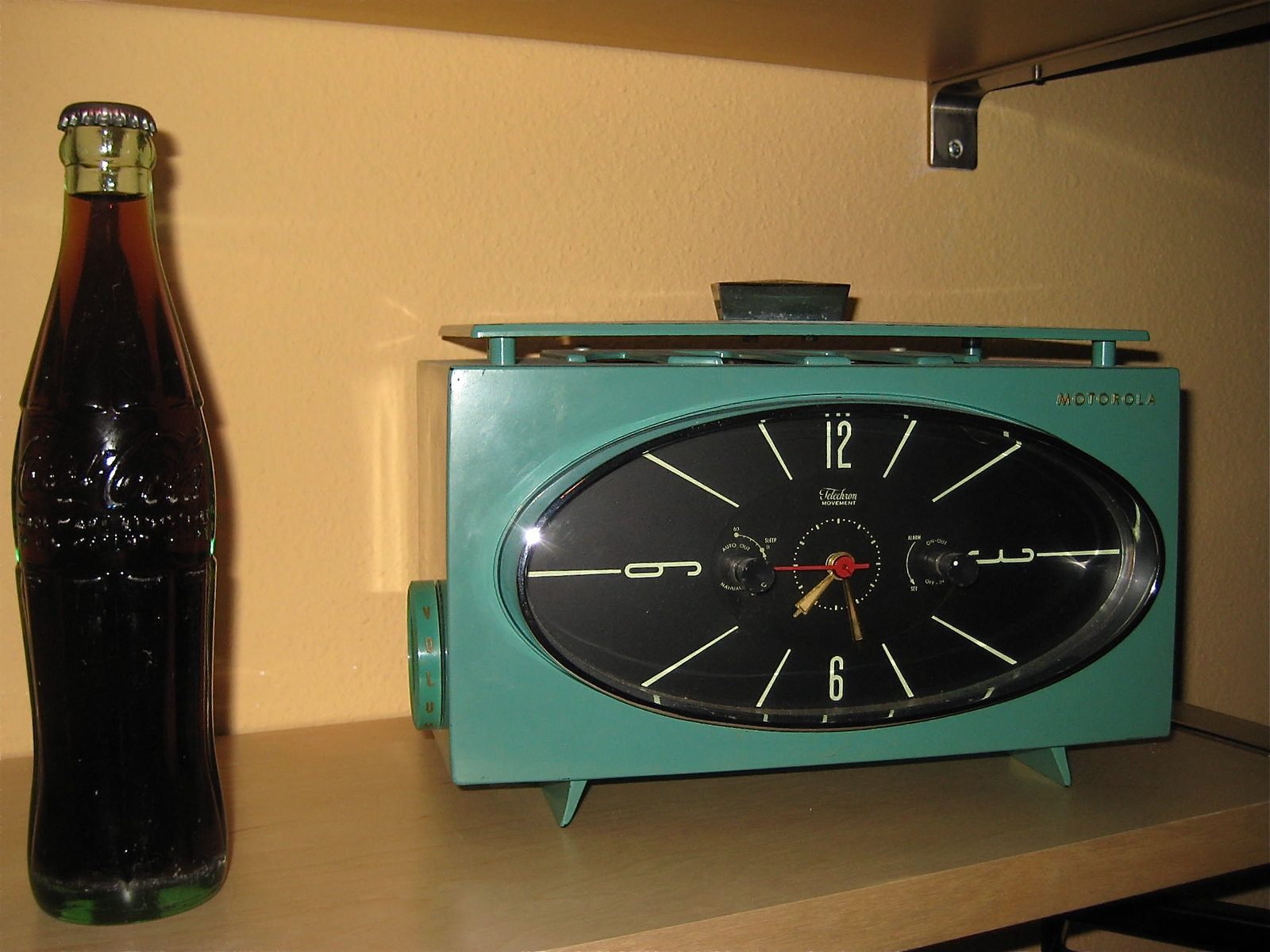In this image, a warm yellow-walled background showcases two wooden shelves. The upper shelf, though partially visible, reveals the bottom edge of its brown wood and a silver metal bracket securing it to the wall. The lower shelf, crafted from light blonde wood, holds two distinct items. On the left, there's a classic glass Coca-Cola bottle filled with the iconic brown soda and capped with silver metal. The curvy bottle features the Coca-Cola name molded into the glass. To its right, a vintage teal Motorola clock radio sits prominently. This rectangular device has a handle on top and a turn dial labeled 'volume' in gold lettering on the left side. The horizontal oval clock face on the front is black, displaying only the numbers three, six, nine, and twelve in off-white. The clock's hands are gold, with a delicate red second hand. The cherished items together evoke a sense of nostalgia on the beautifully lit shelf.